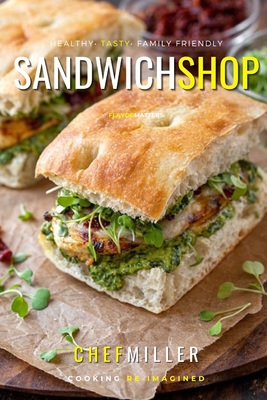The image is a detailed cover of a cookbook titled "Sandwich Shop" by Chef Miller. Boldly highlighted at the top are the words "Healthy, Tasty, Family-Friendly," signifying the book’s focus on wholesome and delicious meals. Near the bottom, the tagline "Cooking Reimagined" is prominently displayed, overlaying a captivating photo. Central to the cover is a mouthwatering sandwich set against the rustic backdrop of brown parchment paper on a wooden cutting board. The sandwich features grilled chicken, avocado, and a pesto spread, topped with fresh green sprouts. It is enveloped in either focaccia or ciabatta bread, making for an appetizing centerpiece. In the background, blurred yet discernible, are additional ingredients and sandwiches, adding layers of culinary intrigue and hinting at the variety within the book.